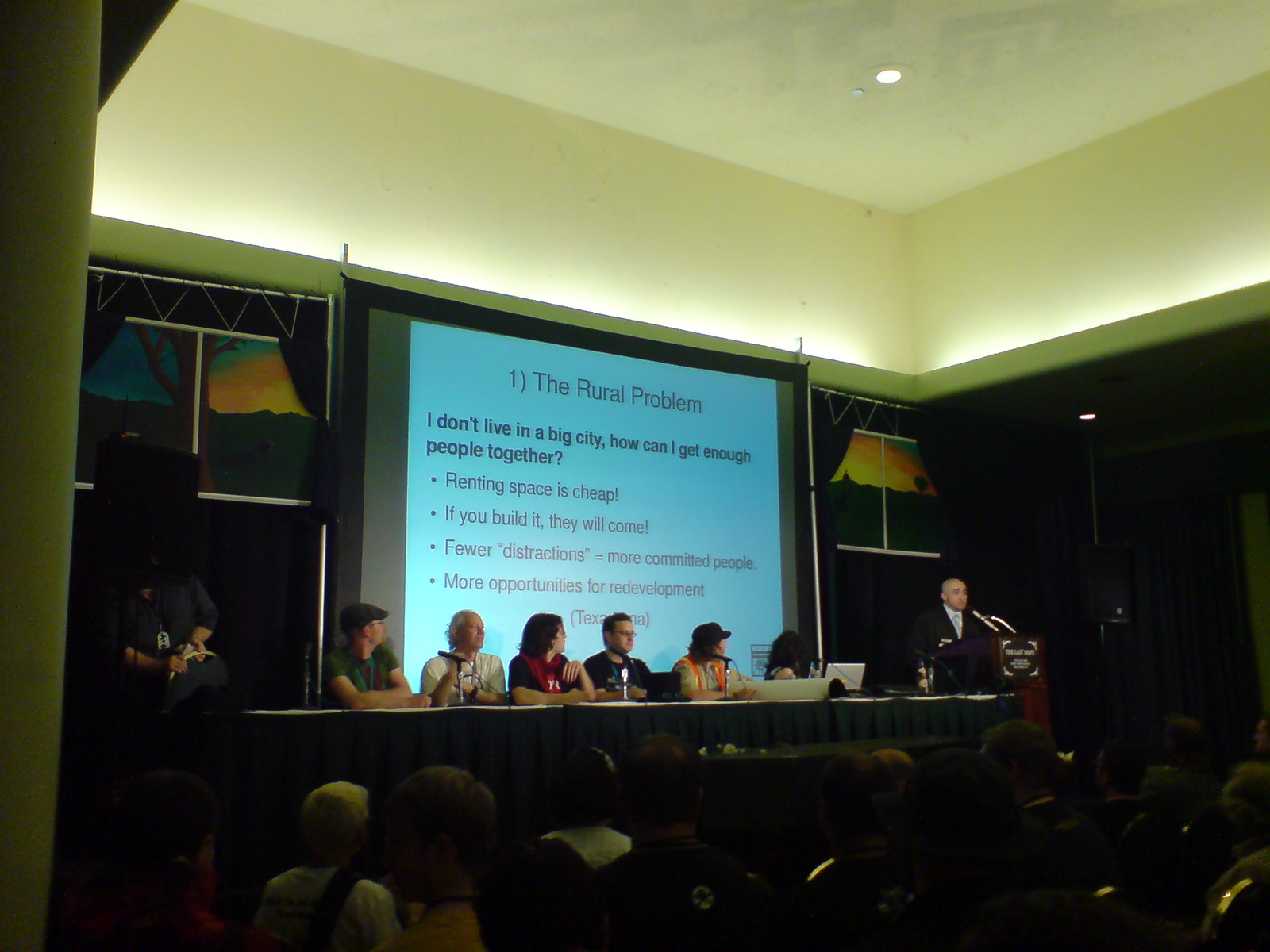The photograph captures a dimly lit conference room, where an engaged audience gazes towards a panel discussion at the front of the room. At a long, cloth-draped table, seven middle-aged speakers face the crowd, one of them actively addressing the attendees. Behind the panelists, a projector screen displays a presentation slide titled "1) The Rural Problem." The slide poses a crucial question: "I don't live in a big city, how can I get enough people together?" It lists several strategic points: "Renting space is cheap," "If you build it, they will come," "Fewer distractions = more committed people," and "More opportunities for redevelopment." The room's ambiance, dim with a sea of faintly visible heads, suggests a sizable turnout, estimated between 20 to 30 people.